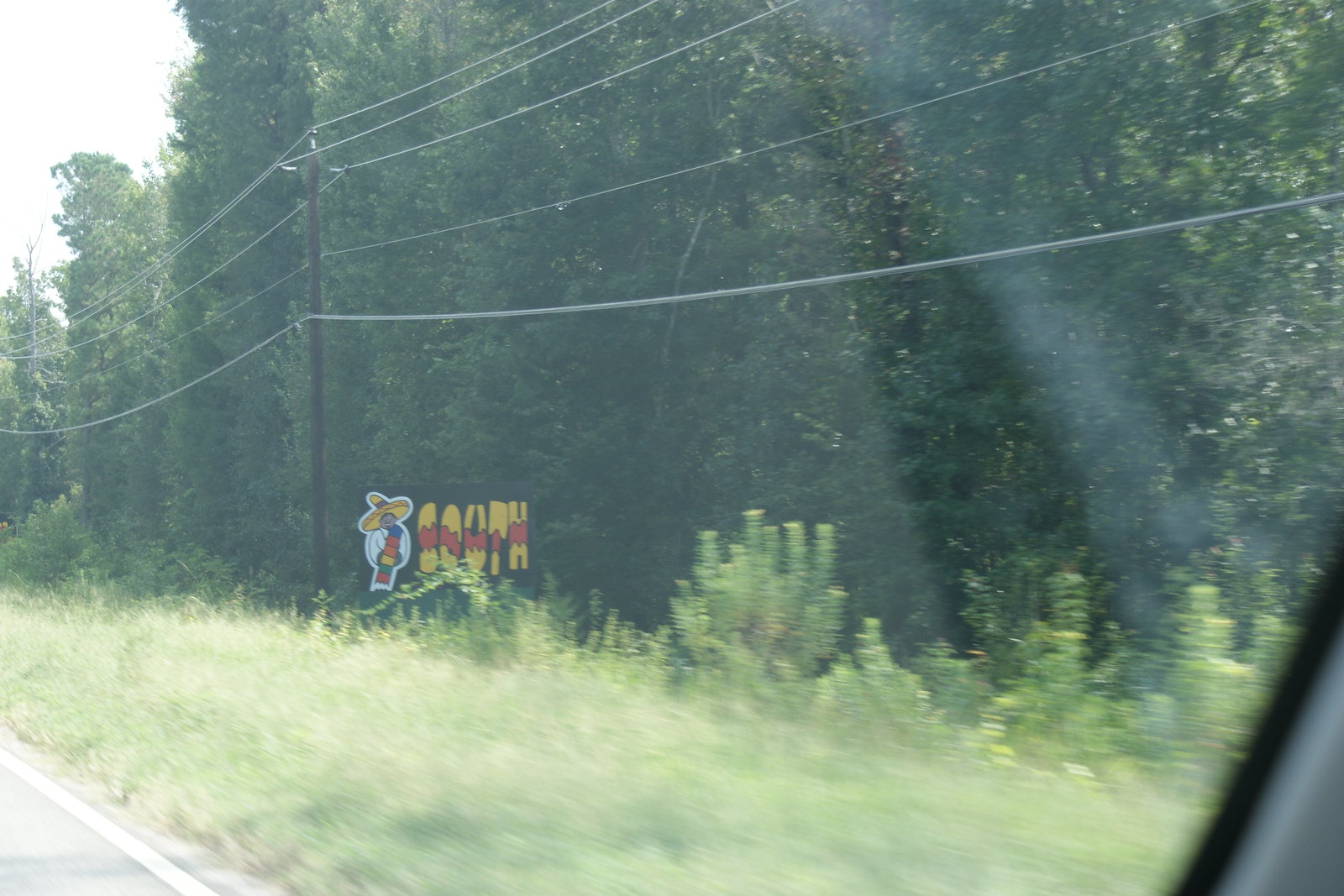Outdoor daytime photograph captured through the right side of a vehicle windshield. The slightly hazy image, affected by the glass and soft focus, features a foreground of wild grass and unkempt weeds. Prominently, just left of center in the lower portion, stands a rectangular black sign with a cartoon Mexican figure donning a sombrero with the word "South" in bold yellow lettering to the right. Adjacent to the sign on the left is a dark brown utility pole supporting six or seven horizontal power lines that extend out of frame to the left. A deep forest backdrop of tall, fully bloomed deciduous trees stretches across the image, indicating a summer setting. The greenery along the front of the tree line and roadside is vivid and lush. The lower left corner shows a small segment of the road marked by a white line, while the lower right corner reveals part of the car window edge and pillar. A sliver of white, cloudy sky peeks through the top left corner, completing the scene.